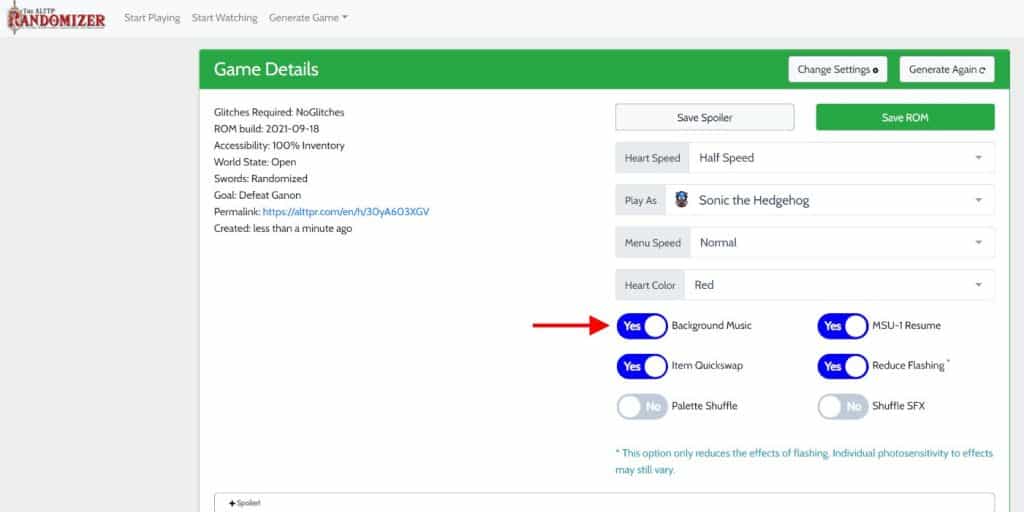The screenshot captures a dynamic webpage related to a game randomizer. The main section of the interface features two distinct rectangles: a larger gray one in the background and a smaller white one that centralizes key information. 

At the top of the smaller rectangle, highlighted in green, are three buttons: "Change Settings," "Generate Again," and "Game Details." The section beneath these buttons is divided into two columns.

On the left side, detailed information about the game configuration is listed:
- No glitches
- ROM build specifications
- 100% inventory
- Open world state
- Randomized swords
- Detailed game-related configurations further listed

On the right side, there's a "Save Spoiler" section where users can save the ROM. A green button also prompts, "Save ROM" — "ROM" being capitalized to denote importance.

Additional interactive options include:
- "Heart Speed" and "Half Speed" buttons
- A drop-down menu labeled "Play as" featuring the name "Sonic the Hedgehog"
- "Menu Speed" set to "Normal"
- "Heart Color" set to "Red"
- Background music enabled, indicated by a red arrow pointing to "Yes"
- "Item Quick Swap," "MSU Resume," and "Reduce Flashing" options all set to "Yes"
- Two additional settings set to "No"

The interface is designed for easy navigation, with clearly marked sections and intuitive controls.